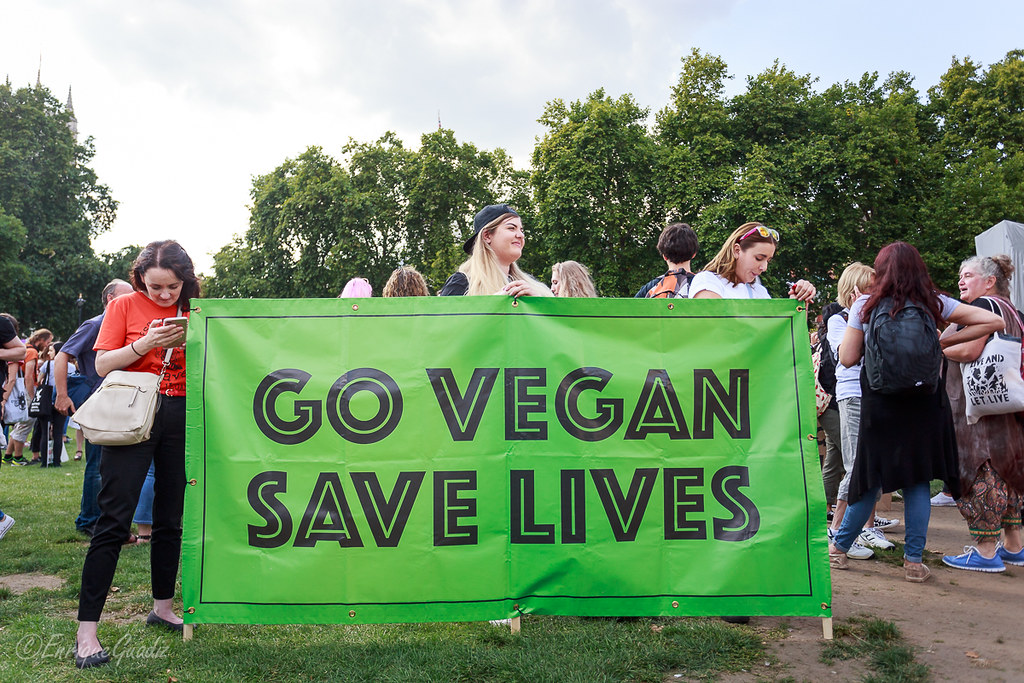In the vibrant midday sun, a large group of protesters gathers in a sprawling green field within what looks like Central Park, as indicated by the towers visible just beyond the tree line to the left. The crowd, comprised predominantly of women, stands against a backdrop of lush trees, creating a serene yet resolute setting for their cause. At the front of this assembly, three determined women hold up a large, eye-catching green tarpaulin sign mounted on wooden posts. The sign, framed by a thin black border, boldly proclaims in large black letters with green outlines, "Go Vegan, Save Lives," with "Go Vegan" on top and "Save Lives" beneath. One woman holding the sign in the center sports a backwards hat and long blonde hair, while the woman on the right has blonde hair adorned with sunglasses perched atop her head. To the left of the sign, a young woman or teenager engrossed in her smartphone and carrying a purse stands out. This scene, possibly marking the beginning or the end of a protest march, encapsulates the spirited and organized advocacy for veganism, surrounded by a diverse and energetic crowd.